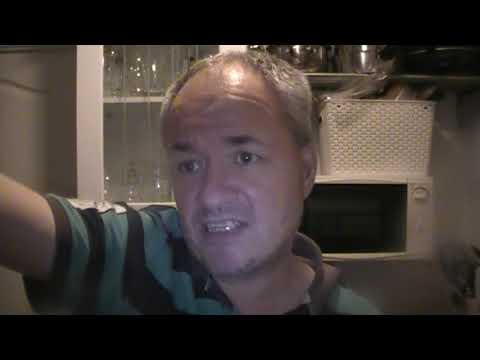This image depicts a middle-aged white man, likely in his late 30s or early 40s, taking a selfie or capturing an image via a webcam. He has a receding hairline with short, graying hair and a scruffy beard with hints of a mustache. His expression is slightly nervous or hesitant, with his mouth partially open, revealing yellowed teeth set in a half-smile. He is dressed in a short-sleeve collared shirt with prominent, thick black and blue-green (or possibly brown) stripes.

The man is positioned in a kitchen, in front of white cabinetry with open shelves. On these shelves, there are various kitchen items including a white microwave or toaster oven, glassware, and some pots or pans. A clear, see-through cabinet door reveals more glassware. Below the cabinets, there is a white mesh basket resting on top of a microwave featuring a black door and control panel. The kitchen wall behind him is white, and the lower right corner of the image is somewhat blurred. The photo appears to be a widescreen shot, indicated by black bars at the top and bottom of the frame.